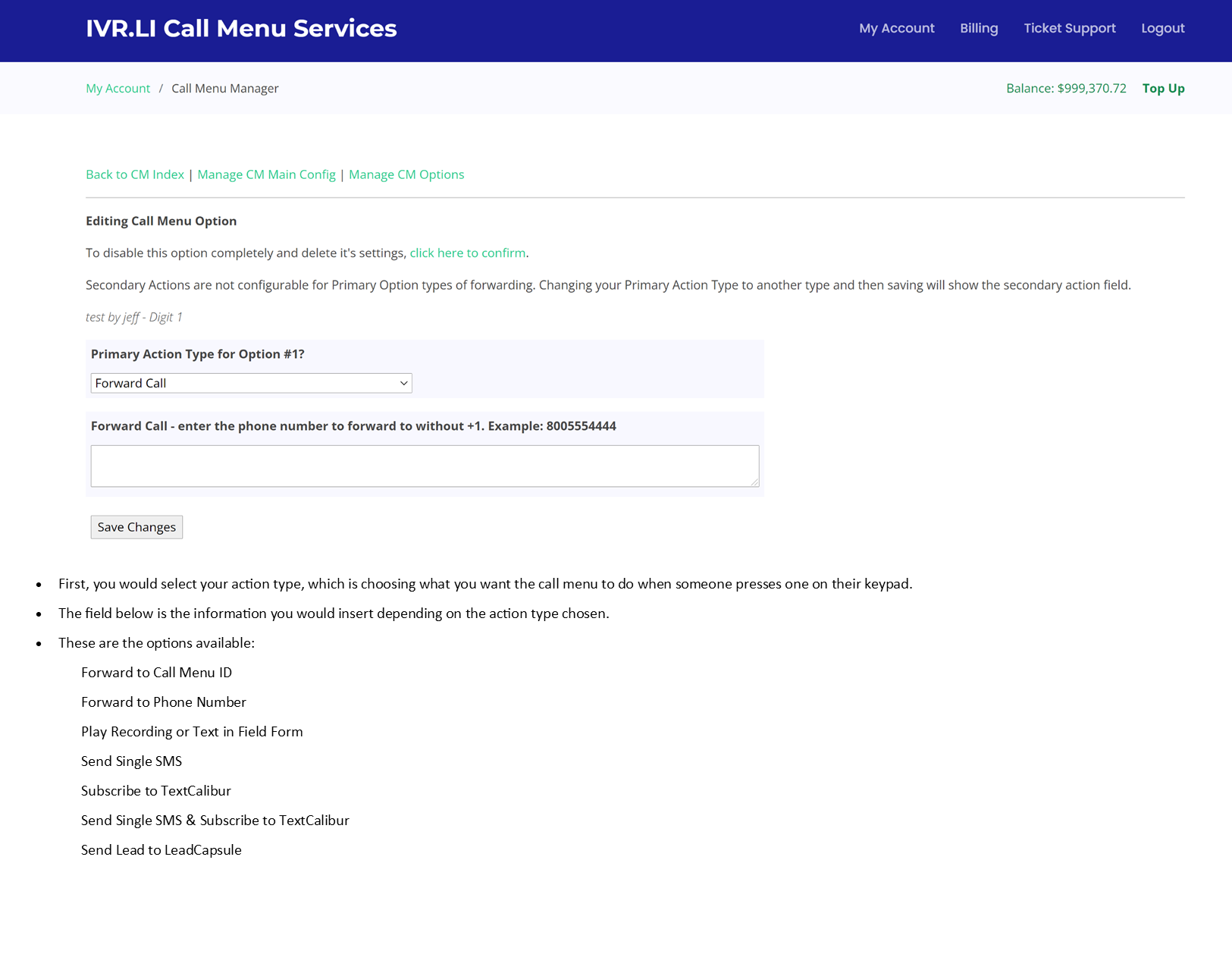The image depicts the user interface of the IVR.LI call menu services, showcasing various account management options and settings for call menu configuration.

At the top of the interface is a blue navigation bar displaying "IVR.LI call menu services." Adjacent to this header, on the right side, are options for "My Account," "Billing," "Ticket Support," and "Logout."

Below the navigation bar, the path indicator reads "My Account / Call Menu Manager." Directly beneath this, the account balance is prominently displayed as $999,370.72, along with a "Top Up" button for adding funds.

Further down, there are several clickable buttons: "Back to CM Index," "Manage CM Main Config," and "Manage CM Options." Below these buttons is a dividing line followed by a section titled "Editing Call Menu Option." Within this section, instructions indicate that to disable and delete a call menu option's settings, the user needs to click a confirmation link.

Additional information notes that secondary actions are not configurable for primary option types designated for call forwarding. It suggests that changing the primary action type and saving the changes will reveal the secondary action field.

The primary action type for option number one is forwarded via a drop-down menu indicating "Forward Call." Beneath this is a field labelled "Phone number to forward to without plus one example," accompanied by a text input box for the phone number. At the bottom of this section is a "Save Changes" button.

The entirety of the interface has a white background, with all the text rendered in black, ensuring clear readability and straightforward navigation.